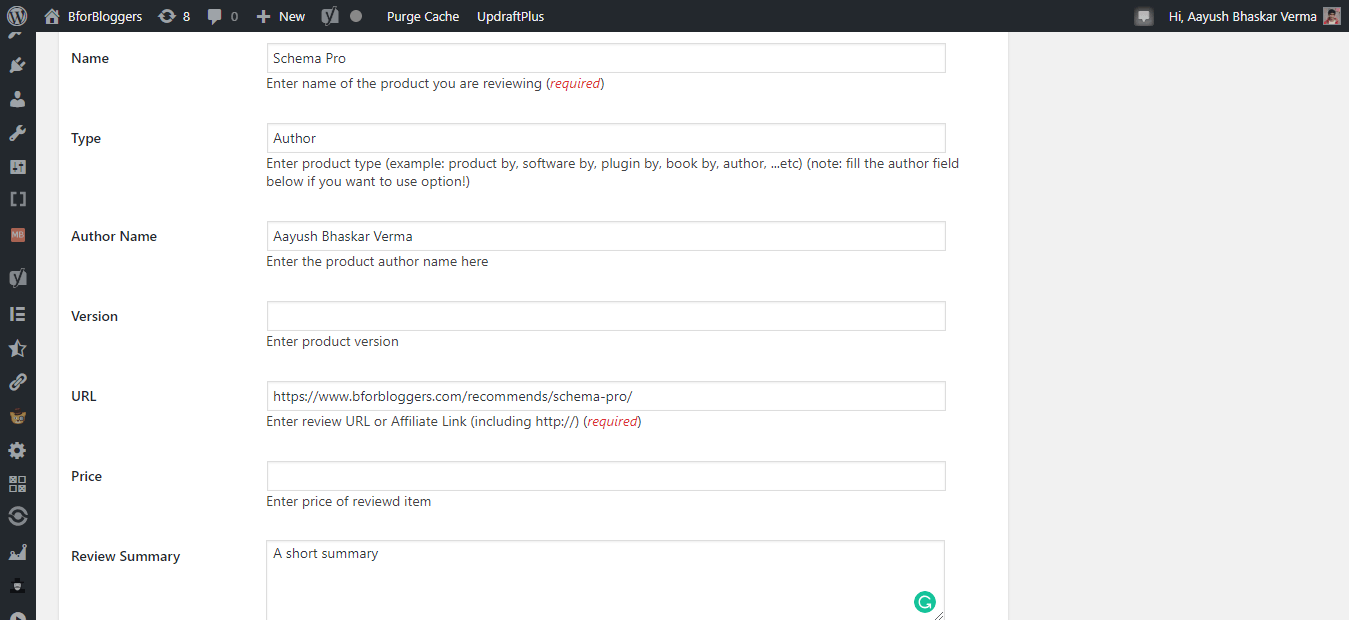Here is a cleaned-up and detailed descriptive caption for the provided image:

---

The image is a screenshot of a WordPress page with a predominantly white theme accentuated by dark blue elements. At the top of the page, a dark blue WordPress bar is visible. On the far left of this bar is the WordPress logo, followed by several buttons: a homepage button labeled "B for bloggers," a share button displaying the number eight, a dimmed comment button with zero comments, a plus button for adding new posts, an unfamiliar 'Y'-shaped symbol, a circle button, a purge cache button, and an UpdraftPlus button. On the far right of the top bar is a message button next to a welcome message that reads, "Hi Ayush Bhaskar Verma," accompanied by a small profile picture in the top right corner.

On the left side of the page, there is a vertical menu bar featuring various icons: an outlet, a person’s profile, a wrench, a settings gear, brackets, and other symbols, representing different navigation options.

The main content area of the page showcases a white survey form. The form fields include:
- **Name:** Instructing the user to enter the name of the product being reviewed, which is filled in as "Schema Pro."
- **Type:** Specified as "Author," indicating the product type.
- **Author Name:** Listed as "Ayush Bhaskar Verma," who is the product's author.
- **Version:** Currently blank.
- **URL:** Providing the full link to Schema Pro.
- **Price:** Currently blank.
- **Review Summary:** Currently blank.

---

This caption provides a detailed description of the elements and layout of the WordPress page captured in the screenshot.